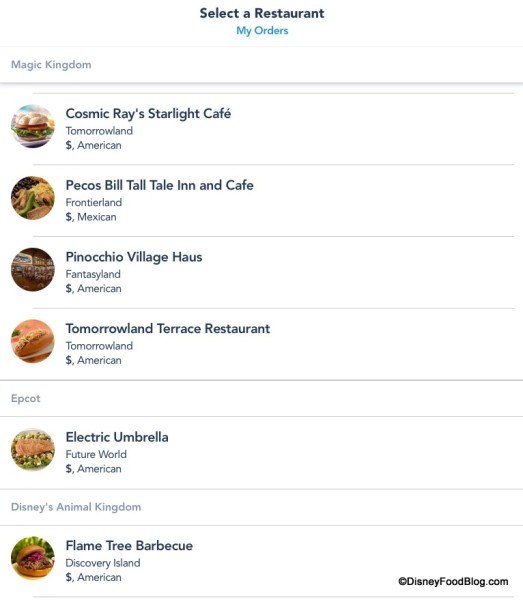The image showcases a webpage from DisneyFoodBlog.com. At the top of the page, the header prominently displays "Select a Restaurant" in a folder named "Print," with both 'Select' and 'Restaurant' capitalized. Beneath this note, in a turquoise color, the menu reads "My Orders," with 'Orders' also capitalized.

Descending the page, the section labeled "Magic Kingdom" appears, followed by a list of four restaurant options, each represented by circles featuring food icons. The listings are as follows: 
1. "Cosmic Ray's Starlight Café"
2. "Pecos Bill Tall Tale Inn and Café"
3. "Pinocchio Village Haus"
4. "Tomorrowland Terrace Restaurant"

Continuing further, the "Epcot" section is highlighted with two dining choices, each accompanied by user icons and food images:
1. "Electric Umbrella"
2. "Disney's Animal Kingdom," which is noted, but it pertains to a restaurant:
   - "Flame Tree Barbecue"

On the left-hand side of the webpage, a copyright notice reads "DisneyFoodBlog.com."